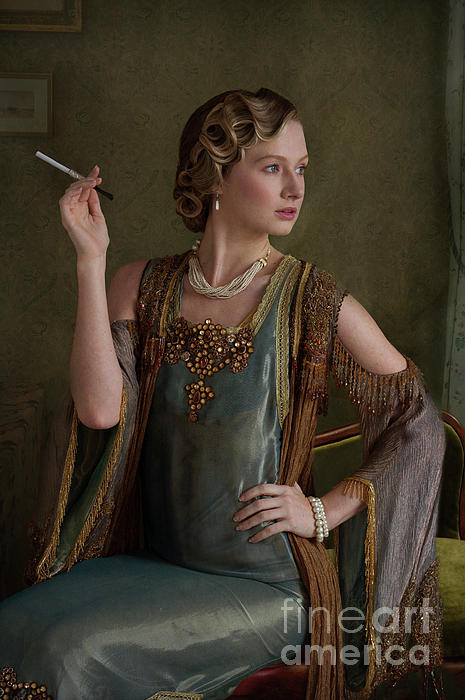This portrait, potentially an oil painting or an AI-generated image, depicts an elegantly dressed woman from the late 1920s or early 1930s. The Fine Art America logo is visible in white in the bottom right corner. The woman, who has a classic finger wave hairstyle known as Marseille, is adorned with multiple strands of pearl jewelry, including a necklace, two bracelets—one larger than the other—and matching dangling earrings. She holds a slender cigarette holder in her right hand. Her attire consists of a green-tinted, satiny dress embellished with gold-colored rhinestones and intricate gold filigree around the neckline and armline. Draped over her shoulders is a beaded shawl in a light purple-gray hue, featuring open sections and ornate beadwork. The woman's left arm rests on her hip, exposing part of her shoulder and upper arm. Seated gracefully in a wooden and upholstered chair, she exudes the poised aura of a socialite, set against a simple, beige background wall that underscores her sophisticated appearance.